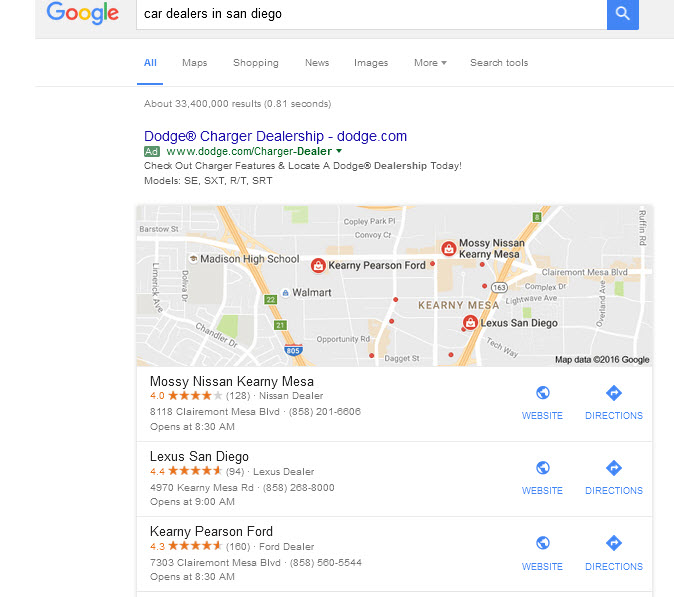Screenshot of a Google search for "black car dealers in San Diego." At the top, the familiar multicolored Google logo (blue, red, yellow, green) appears on a thin gray bar. Below, the search query is displayed in a blue text box with a magnifying glass icon. Tabs for "All," "Maps," "Shopping," "News," "Images," "More," and "Search tools" are visible, with "All" highlighted with a blue line underneath. 

The search results section shows the number of results and the time taken for the search. The first result is an advertisement for "Dodge Charger dealership" on Dodge.com, indicated by green 'Ad' text. Below, a gray Google Maps image displays various dealership locations in San Diego, marked by green, blue, and red icons. The map includes dealership names like Kearny Pearson Ford, Mossy Nissan, and Kearny Mesa Lexus.

The listings below the map provide detailed dealership information:
1. **Mossy Nissan Kearny Mesa**: 
   - Rated: 4.0 stars from 128 reviews 
   - Type: Nissan dealer 
   - Address: 8118 Clairemont Mesa Boulevard
   - Phone: 858-201-6606
   - Opens: 8:30 AM
   - Options: Website, Directions

2. **Lexus San Diego**:
   - Rated: 4.4 stars from 94 reviews 
   - Address: 4970 Kearny Mesa Road
   - Phone: 858-268-8000
   - Opens: 9:00 AM
   - Options: Website, Directions

3. **Kearny Pearson Ford**:
   - Rated: 4.3 stars from 160 reviews 
   - Address: 7303 Clairemont Mesa Boulevard
   - Phone: 858-560-5544
   - Opens: 8:30 AM
   - Options: Website, Directions

At the bottom, copyright information reads "map data, copyright 2016, Google."